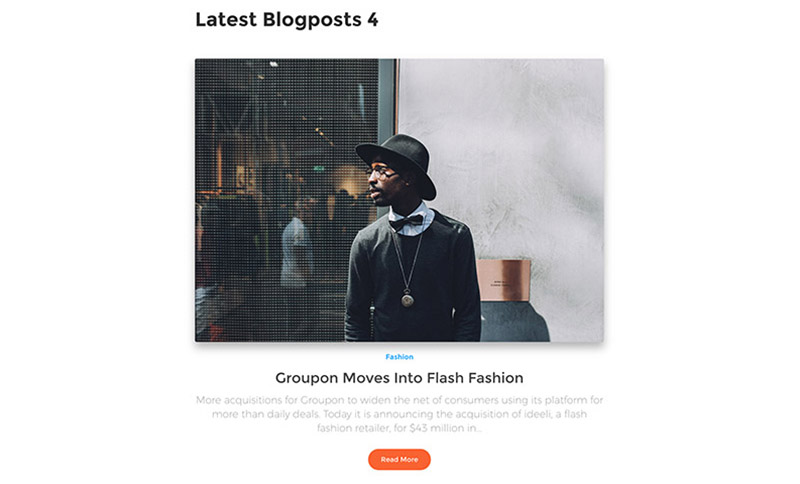**Descriptive Caption:**

In this promotional image with a white background, the headline "Latest Blog Post" is prominently displayed at the top in large black bold letters. The image itself is square and centrally features a well-dressed man. He is wearing a gray sweater, a gold necklace that hangs past his chest, a white collar, and a black bow tie. The man, who has dark skin, is also wearing eyeglasses and a black hat. His gaze is directed to the left side of the image.

Behind him, there is a gray wall on the right side, leading down to a gray table that supports a cardboard box by his arm. On the left side of the image, the background reveals the interior of a store, separated by a gray metal grid-like fence. Inside the store, there's a man in a white shirt walking, shelves stocked with clothes, dim ceiling lights, and some art, indicating a fancy retail environment.

Centered below the square image, the word "Fashion" is written in blue text. Further below, the caption reads: "Coupon moves into flash fashion" in black letters, followed by a more detailed explanation stating, "More acquisitions for Coupon to widen the net of consumers using its platform for more than daily deals. Today it is announcing the acquisition of Idealy, a fast-fashion retailer, for $43 million..." The text trails off with an ellipsis, and an orange "Read More" button invites viewers to learn more.